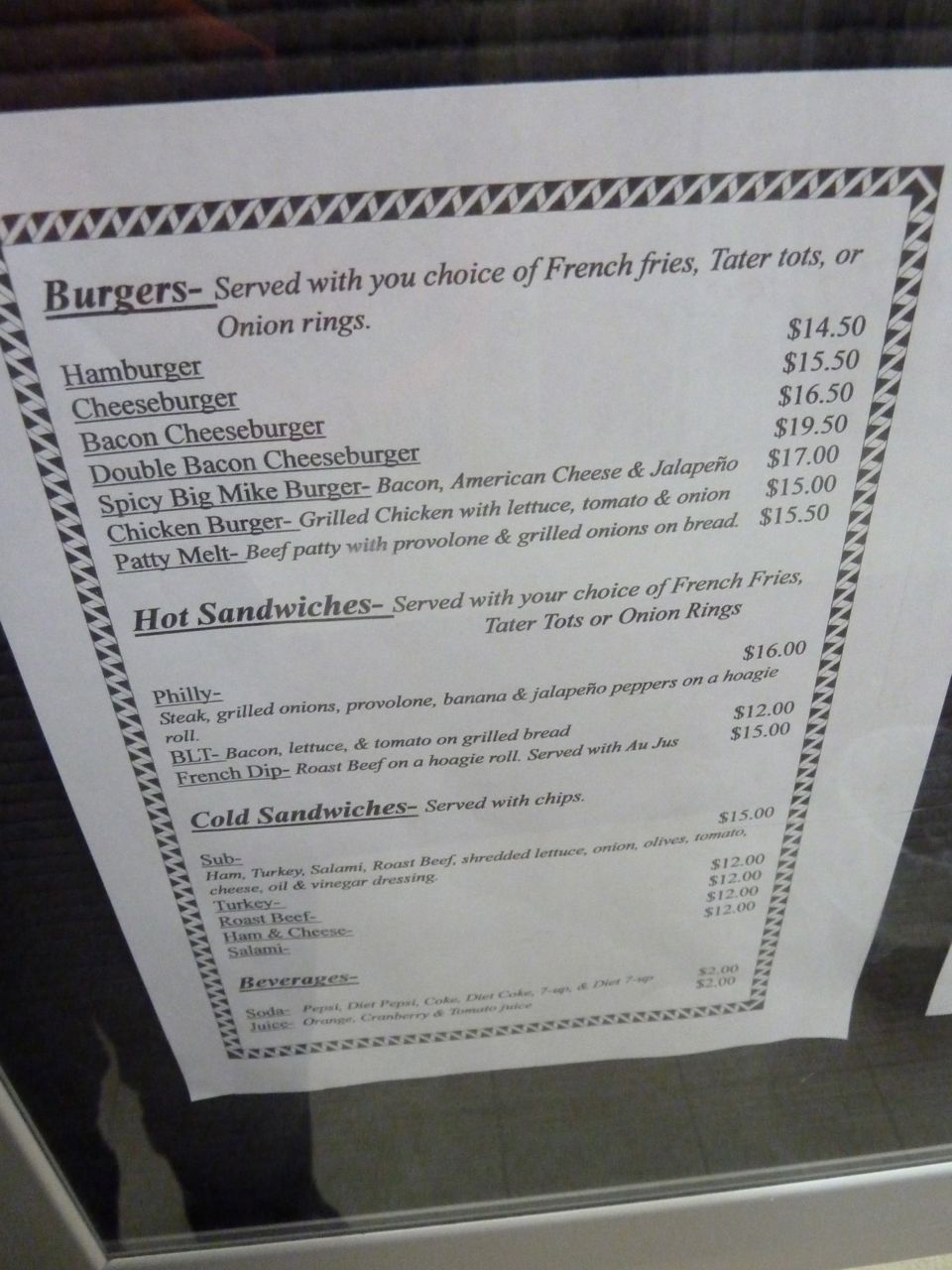Here's a detailed and cleaned-up caption for the image:

---

The photo captures a black and white menu, neatly framed in black and prominently displayed on a piece of paper. A shadow of a person is visible in the mirror where the menu is posted. The menu lists the following items:

**Burgers** (all served with a choice of French fries, tater tots, or onion rings):
- **Hamburger:** $14.50
- **Cheeseburger:** $15.50
- **Bacon Cheeseburger:** $16.50
- **Double Bacon Cheeseburger:** $19.50
- **Spicy Baked Mike Burger:** Bacon, American cheese, and jalapeno - $17.00
- **Chicken Burger:** Grilled chicken with lettuce, tomato, and onion - $15.00
- **Patty Melt:** Beef patty with provolone and grilled onions on bread - $15.50

**Hot Sandwiches** (all served with a choice of French fries, tater tots, or onion rings):
- **Philly Cheesesteak:** Steak, grilled onions, provolone, banana, and jalapeno peppers on a hoagie roll - $16.00
- **BLT:** Bacon, lettuce, and tomato on grilled bread - $12.00
- **French Dip:** Roast beef on a hoagie roll served with au jus - $15.00

**Cold Sandwiches** (all served with chips):
- **Sub Sandwich:** Ham, turkey, salami, roast beef, shredded lettuce, onion, olives, tomato, cheese, and oil and vinegar dressing - $15.00
- **Turkey Sandwich:** $12.00
- **Roast Beef Sandwich:** $12.00
- **Ham and Cheese Sandwich:** $12.00
- **Salami Sandwich:** $12.00

**Beverages:**
- **Soda:** Options include Pepsi, Diet Pepsi, Coke, Diet Coke, 7Up, and Diet 7Up - $2.00 each
- **Juice:** Options include orange, cranberry, and tomato juice - $2.00 each